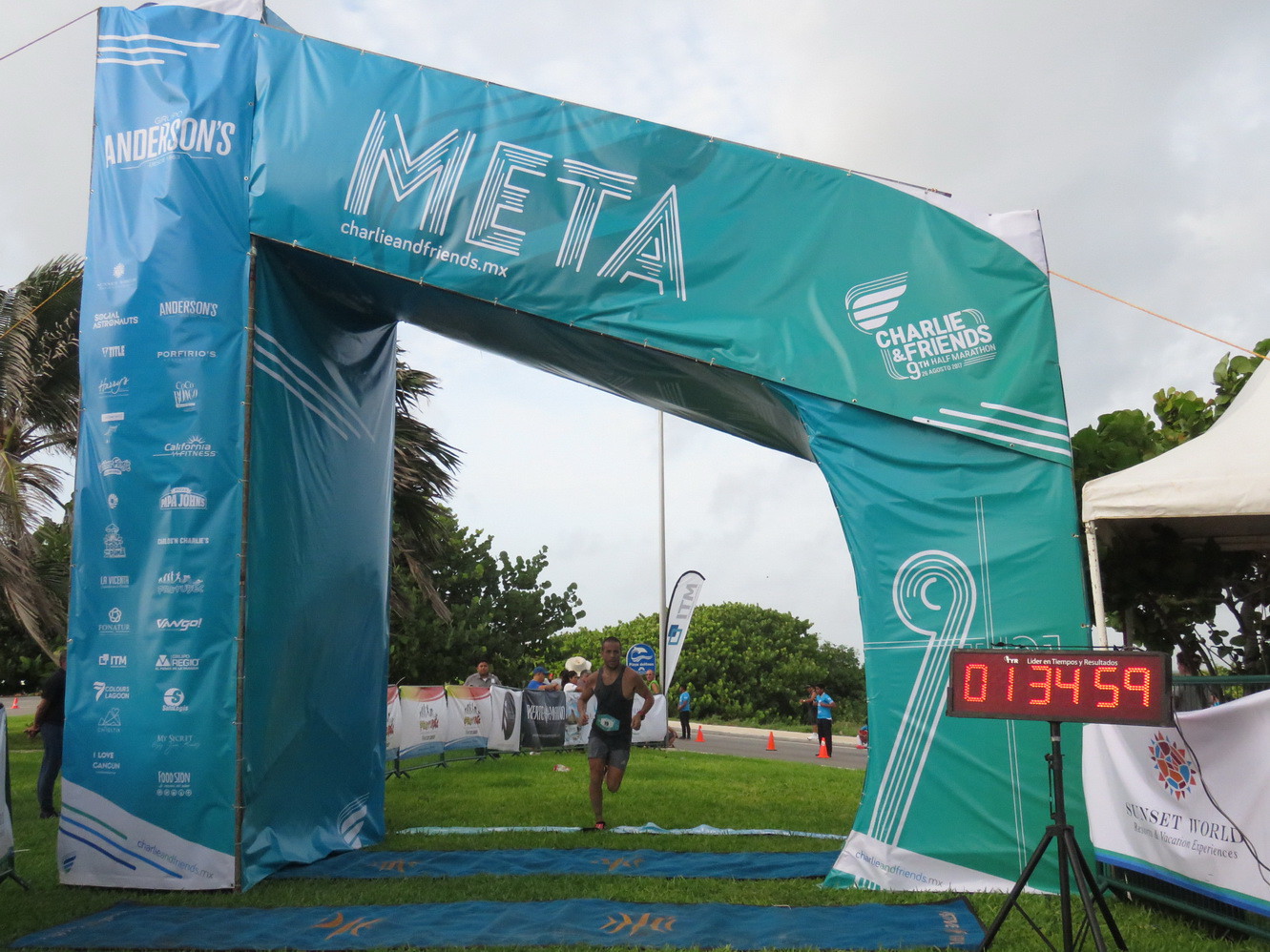The image captures a vibrant scene of a race event on a cloudy day with a gray and white sky. At the center is a large, partially tilted, balloon-like arch, predominantly blue with "Meta" in large white letters on top and "charlieandfriends.mx" on the right. The arch spans a grassy area, with a blue tarp on the ground beneath it, and leads to a street set with orange cones. A runner in a black T-shirt and gray shorts is in the middle of crossing the finish line, marked on the grass. To the right of the arch is a digital timer displaying "01:34:59" on a tripod. Banners with "Sunset World" and other advertisements adorn the railing to the left, creating a festive atmosphere. Observers in blue shirts stand along the sidewalks and street, lined with green leaf trees and some palm trees on the far left. The scene buzzes with activity, capturing the energy of the racing event.